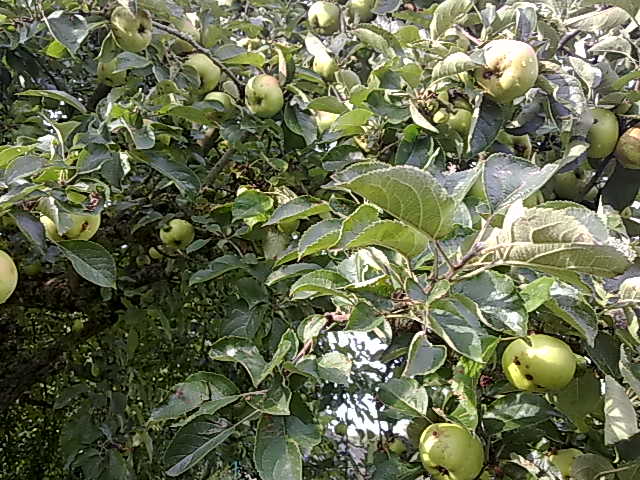This photograph captures a somewhat close-up view of a dense mass of greenery, likely within an orchard or garden. Large, serrated green leaves dominate the image, offering substantial coverage, casting shadows at the bottom left of the frame that accentuate the sunlight filtering through from above. The plants, heavily adorned with fruit, showcase numerous green tomatoes—or possibly green apples—hanging from various stems and branches. These fruits, numbering between 12 to 20, exhibit a consistent light green hue with some displaying water droplets, particularly where the sunlight glints off their surface in the top right corner of the image. The overall scene reflects a bright, sunny day with light streaming through the foliage, creating a natural, softly dappled effect.